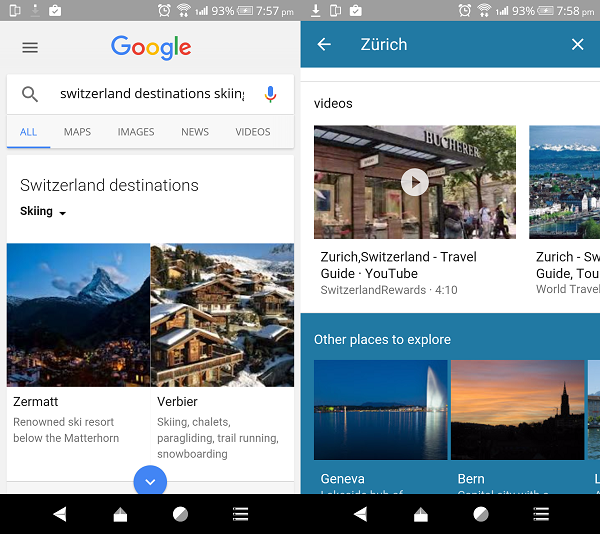The image features a pair of screenshots from an Android device displayed side by side. The left screenshot shows a Google search results page for the query "Switzerland destinations skiing." The search bar is located at the top, with menu options below it including All, Maps, Images, News, and Videos. Under this menu, there is a dropdown that can be switched, currently set to show "Switzerland destinations skiing." Following this, there are two sections: the first features an image and text description of Zermatt, a renowned ski resort situated below the Matterhorn. The second section highlights Verbier, known for its skiing, chalets, paragliding, trail running, and snowboarding.

The right screenshot focuses on Zurich, featuring a video result from YouTube with the title "Zurich, Switzerland Travel Guide." The video's thumbnail is partially visible, and the title appears to the right, though it is mostly cut off. Below this, there is a prompt on a blue background suggesting other places to explore, specifically Geneva and Bern.

The visual presentation effectively illustrates detailed information about skiing destinations in Switzerland, highlighting specific locations and available media resources.